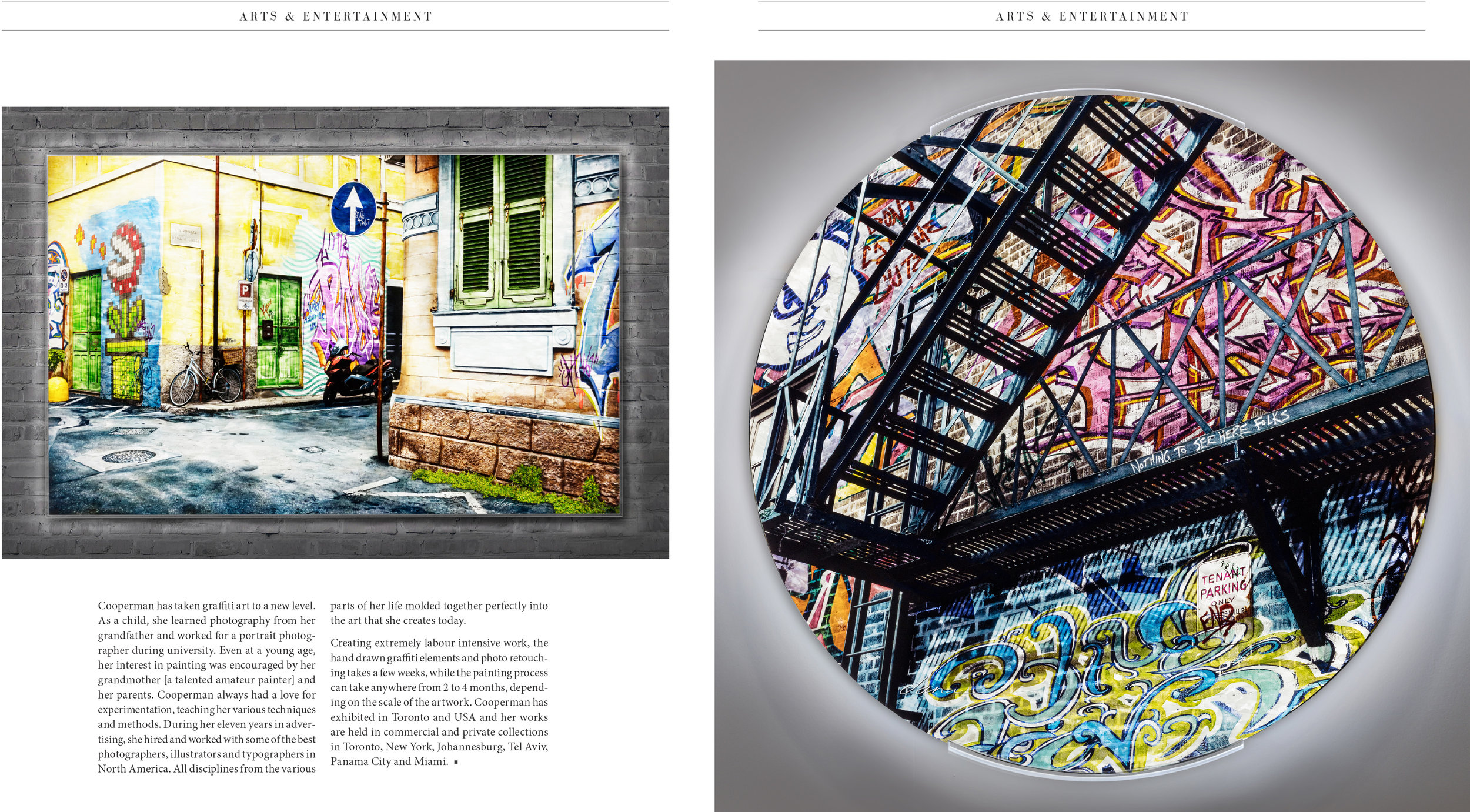This image features a magazine spread highlighting the graffiti art of Cooperman. The layout includes two richly detailed pictures of urban scenes with heavily graffitied walls. The left picture shows two buildings adorned with graffiti, the most notable being a vibrant piranha plant from the Mario series emerging from a green pipe on the left building. Other details include a real bicycle, a green door, and a blue street sign with an upward white arrow. The right picture showcases a black fire escape against a wall covered in graffiti. A white face with a blue outline stands out in the upper left corner, and below the fire escape, a tenant parking sign is also decorated with graffiti.

Above both images, "arts and entertainment" is elegantly displayed in fancy text. Accompanying the visuals, the article delves into Cooperman's background, highlighting her early influences from her grandfather's photography and her grandmother's painting. Her career in advertising, spanning 11 years, honed her skills with top photographers, illustrators, and typographers. Known for creating labor-intensive pieces, Cooperman's hand-drawn graffiti elements and photo retouching take weeks, while the painting process can span two to four months. Her work has been exhibited in Toronto, the USA, and is part of various collections across the globe, including New York, Johannesburg, Tel Aviv, Panama City, and Miami.